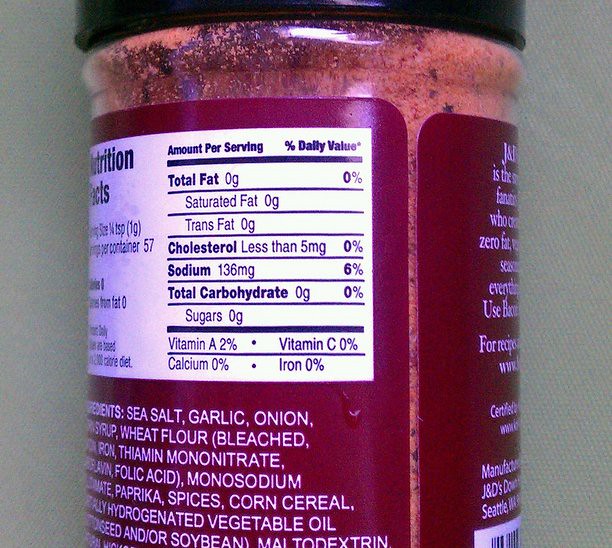This image features a close-up view of a spice bottle placed against a subtly textured, white background, possibly a napkin. The bottle is round with a barely visible black lid. Its label predominantly showcases a reddish-maroon hue with a white box containing the nutrition facts. The bottle houses a finely ground spice, evident from its brownish-reddish color. The text on the label is somewhat visible, listing ingredients such as sea salt, garlic, onion, syrup, wheat flour (bleached), iron, thiamine mononitrate, folic acid, monosodium, paprika, spices, corn cereal, and hydrogenated vegetable oil.